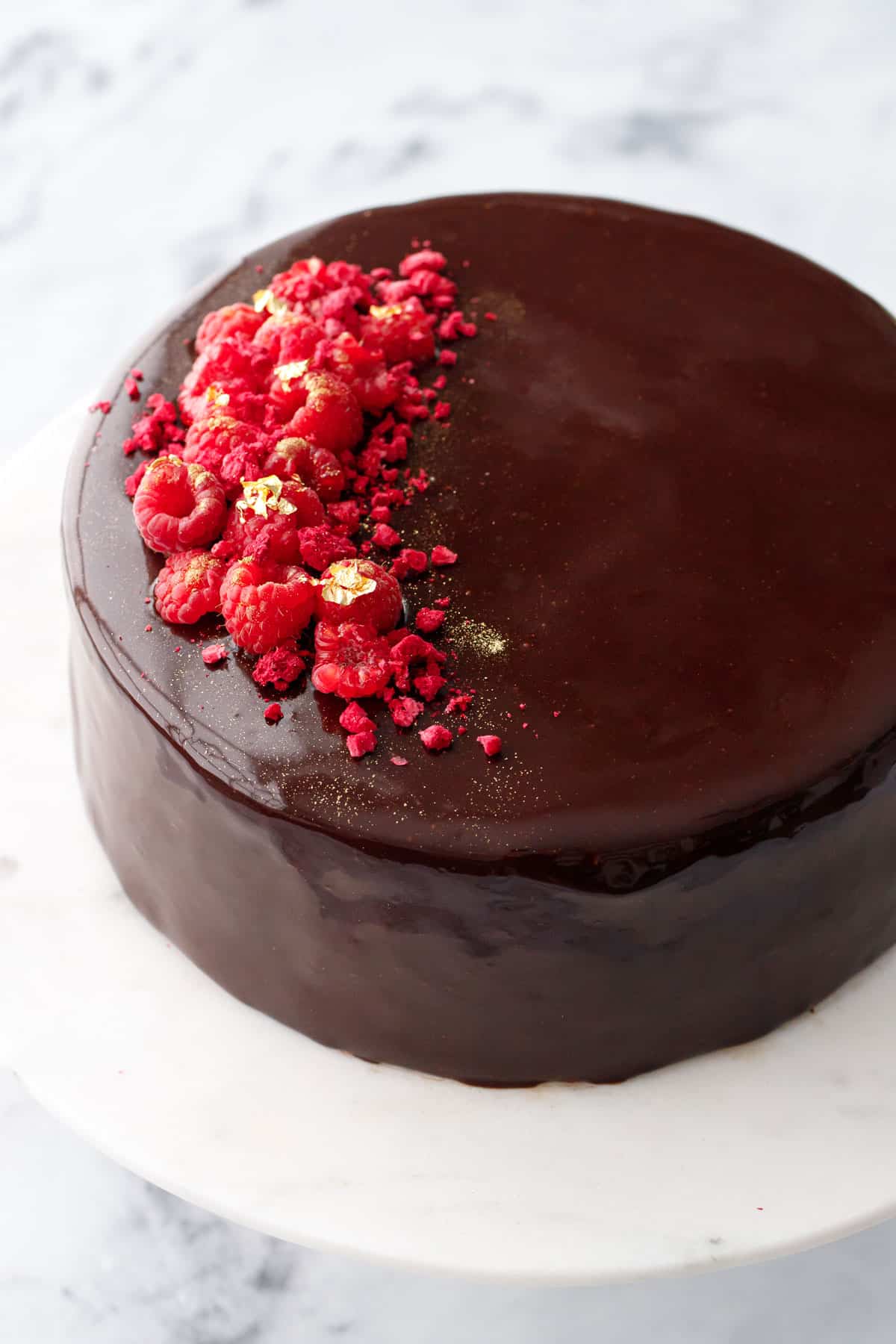This photograph showcases a round, gourmet dark chocolate cake, elegantly positioned on a pristine white pedestal or plate. The rich, dark brown layers of the chocolate cake are coated with a dark icing, creating a sumptuous, sleek appearance. The top of the cake is adorned with a generous spread of vibrant red raspberries, which cover approximately a third to half of the dessert, adding a pop of color and a hint of tartness. Some sprinkles of berry pieces might also be seen enhancing the visual appeal. The entire setup rests on a sophisticated, grayish-silver granite or marble-like table, creating a refined backdrop that accentuates the cake's decadent presentation. This delectable creation, possibly a centerpiece at a bakery display or a festive gathering, exudes a sense of homemade artistry while appealing to anyone with a taste for gourmet pastries.